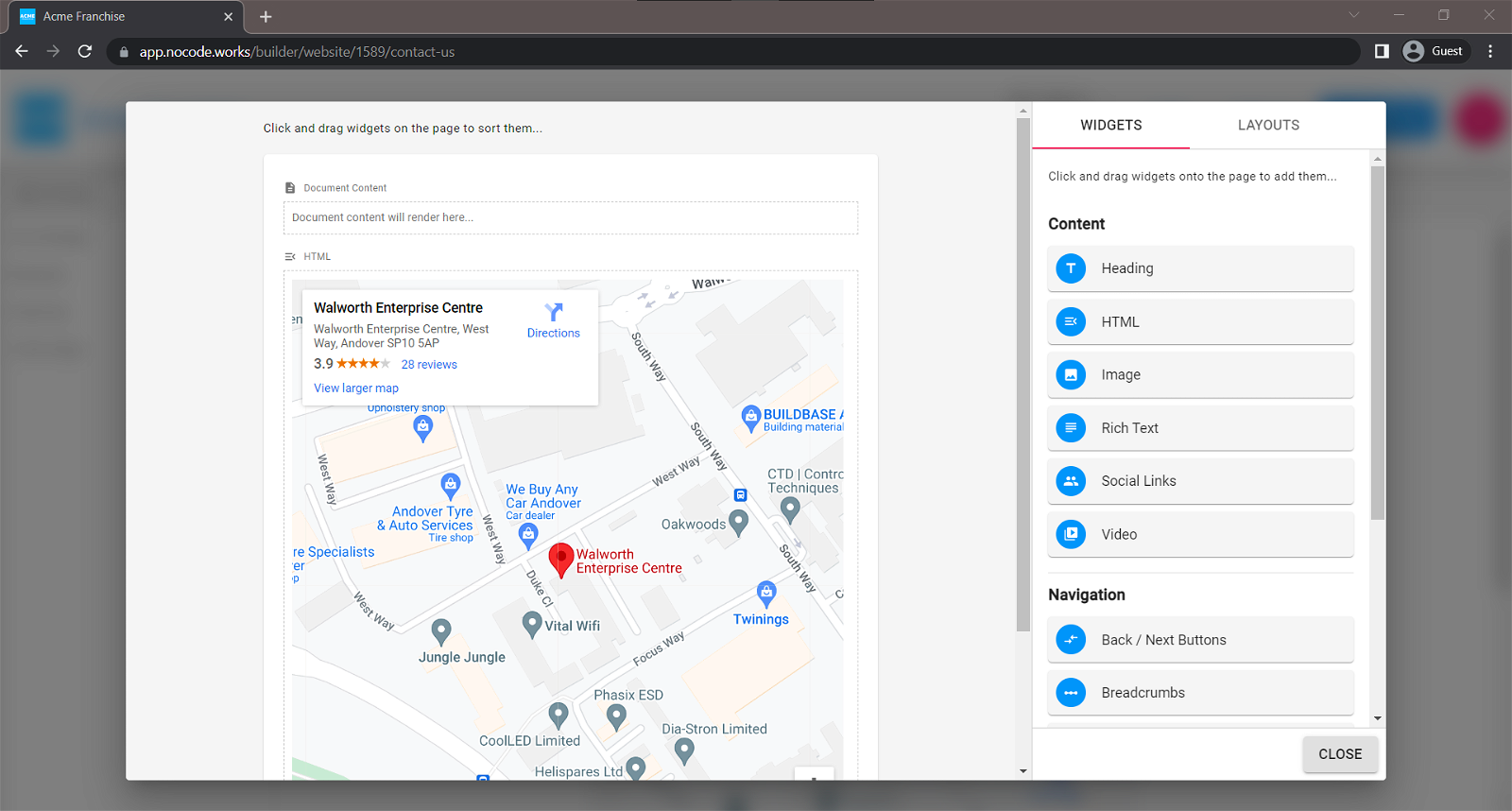Image Description: 

The image appears to depict a computer screen displaying a map application or webpage interface. The background is a dark gray color, framing a larger, lighter gray rectangular box in the center of the screen. At the top, there's a darker gray bar resembling a browser tab bar, featuring a blue icon that is not clearly legible. 

Directly below this is a browser-like bar, showing an icon of a person labeled "Guest" on the left side and three vertical dots on the far right corner, indicating more options.

Dominating the central part of the screen is a map interface, seemingly from a tool like Google Maps or a similar navigation service. The map displays the location of "Walworth Enterprise Center" and nearby landmarks such as "Walworth Enterprise Center West." Additional details include acronyms like "WAG," "Amber," and "SPF or SP10 SAP," along with a rating of 3.9 stars based on 28 reviews. There is also a "View larger map" link, and a directions button featuring an arrow pointing up and to the right.

On the right side of the screen, a vertical toolbar lists several clickable buttons labeled "Widgets," "Layouts," "Content," "Heading," "HTML," "Image," "Rich Text," "Special Links," and "Video." These appear to be tools for customizing or interacting with the content displayed on the screen.